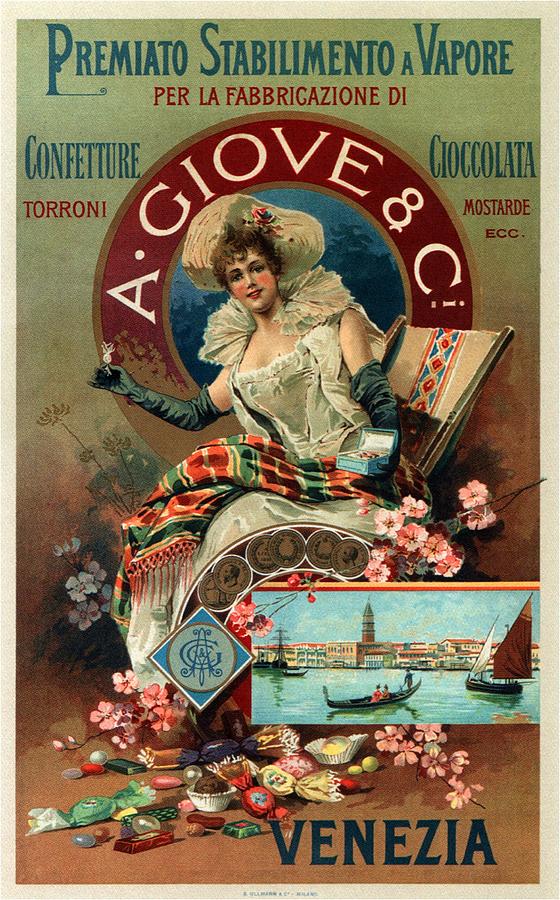An old-fashioned poster showcases a vintage lady elegantly dressed in period attire. She has short, curly hair topped with a stylish hat. Her white dress, featuring a high, outward-standing collar, falls long and gracefully around her. The dress is intricately designed with a low neckline and short sleeves. Her arms are adorned with long, green, silky gloves extending past her elbows.

In her left hand, she holds a small, blue box, while her right hand clutches what appears to be a piece of candy. Draped across her lap is a multicolored striped blanket in shades of orange and green, fringed at the edges. The chair she is seated on features a matching design, reminiscent of an Indian pattern, with a beige base adorned with coins or medals, six in total, overlapping along a curved line.

A blue diamond-shaped medallion with a round center and a central symbol adds to the ornate details. To the right side of the poster, there is an illustration of a lake with buildings and boats, suggesting a serene outdoor scene. The ground around the woman is scattered with treats such as candies, flowers, and possibly cookies.

Prominent text in capital letters reads "Phoenicia" on the right side. The top of the poster carries an inscription in a different language in blue, flanked by red text below it. Additional words appear on the left and right sides, similarly formatted with blue and red text beneath.

Behind the woman, a round backdrop features the text "A.GIOVENC" in a gold-trimmed, blue background, adding a final touch to this intricate and detailed illustration, reflecting an old-world charm.